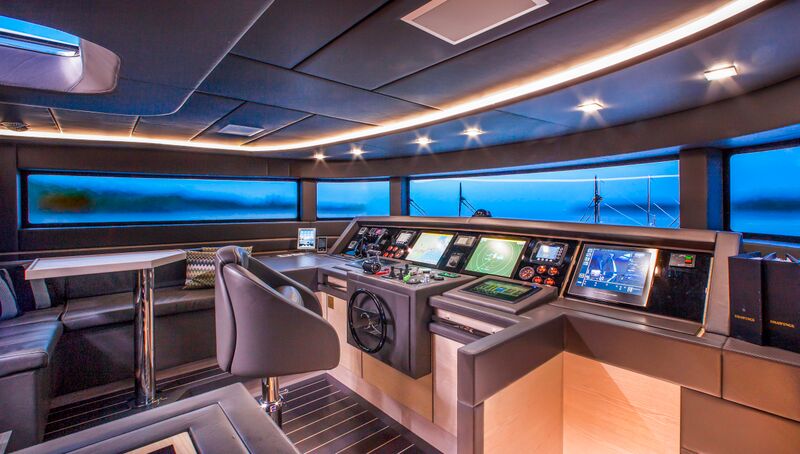This detailed photograph captures the interior of the captain's area on a large private yacht or sophisticated vessel, distinctly angled to showcase its layout. Dominating the center of the room is a single green captain's chair positioned behind a black steering wheel. Above the wheel, a comprehensive array of instruments, toggles, and buttons is arranged, offering control over the ship's numerous functions. Multiple display screens with white, green, and blue hues are spread mostly across the center and towards the right side of this control panel.

A band of slender glass windows stretches from the middle left to the middle right of the image, offering limited but crucial visibility to the exterior. Above these windows, lighting embedded in a segmented gray padded ceiling illuminates the space. On the floor beneath the control panel, white cabinets sit before a black and gray floor adorned with parallel white lines.

To the bottom left-hand corner of the image, a white table supported by a chrome pole is visible, accompanied by gray seating, adding a touch of luxury to the utilitarian setting. Overall, the expansive cockpit, combined with its detailed control layout and plush design elements, signifies the high level of sophistication expected in a private yacht's control room.